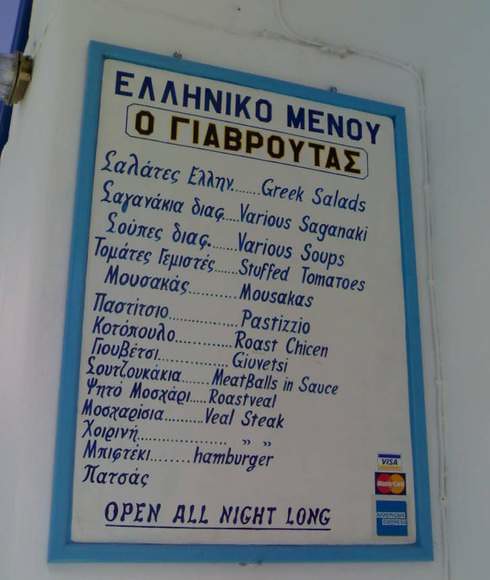This image depicts a menu sign for a restaurant, likely located in a tourist area of Greece, as evidenced by the bilingual display in both Greek and English. The menu, bordered and inscribed in blue on a white background, is affixed to a wall, presumably outside the restaurant. The bottom right corner showcases stickers indicating payment acceptance of Visa, MasterCard, and American Express. The menu declares "Open All Night Long" at the lower section.

In total, there are 14 listed menu items, with the left side featuring the Greek names and the right providing English translations. The offerings include:

1. Greek Salads
2. Various Saganaki
3. Various Soups
4. Stuffed Tomatoes
5. Moussakas
6. Pastisio
7. Roasted Chicken
8. Gouvesti
9. Meatballs and Sauce
10. Roasted Veal
11. Veal Steak
12. Hamburger

Note: The last two items are not translated into English.

The image is a close-up, limiting visibility to just the menu itself without any additional context or surroundings of the establishment.